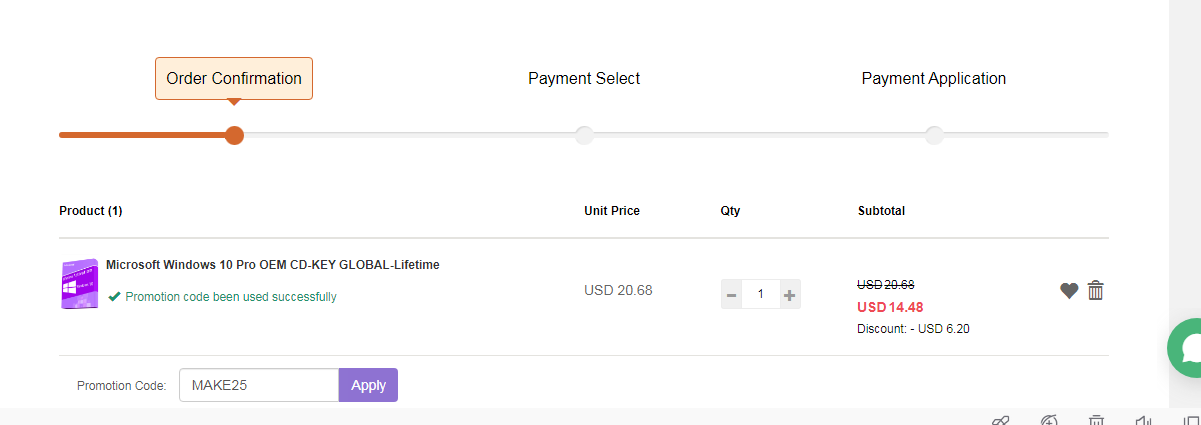**Descriptive Caption:**

The image is a detailed screenshot from a website's order page, lacking both its header and footer. The background is predominantly white, accented with a thin gray line at the top that transitions to an orange color on the left side. A prominent circle and a pink rectangle with the text "Order Confirmation" indicate the page is tracking a user's payment process. The progress is further illustrated with markers: "Payment Select" centered at the top and "Payment Application" on the far right.

Below this progress bar, the product description is displayed: "Microsoft Windows 10 Pro OEM CD-Key Global Lifetime." To the left of this description, a small purple square showcases the Microsoft Windows logo, symbolizing the product.

A blue note indicates that a promo code has been successfully applied. Central to the page, under the "Unit Price" section, the price is listed as USD $20.68. The quantity is specified as one. Notably, a discount price is highlighted below in red, showing a reduced cost of USD $14.48.